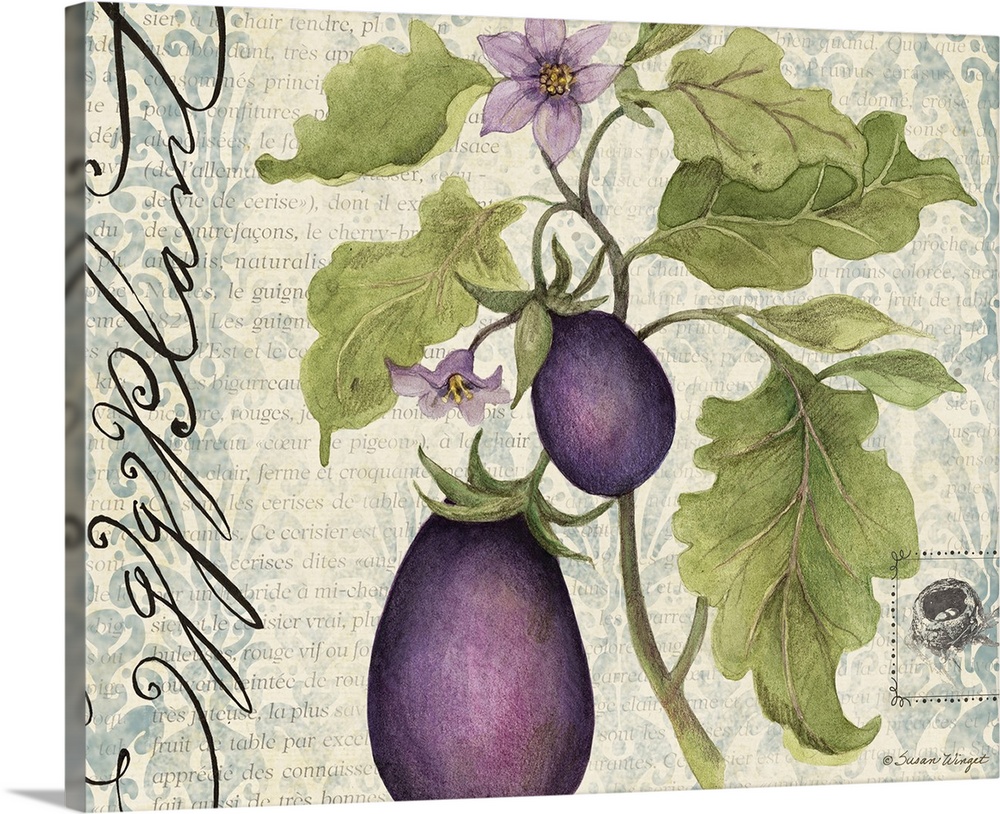This image displays a sophisticated canvas art print set upright against a white-and-black background, casting a faint shadow to its left. The print itself resembles aged yellow paper, overlaid with light gray, slightly transparent text that gives the impression of being antique or from a foreign language document. The background text is interspersed with greenish, abstract floral and leaf designs that add to the vintage aesthetic.

The primary focus of the artwork is a detailed depiction of an eggplant plant. The plant features numerous large, veined leaves and two prominent dark purple eggplants situated in the lower half. Above these vegetables, two light purple eggplant flowers with vivid yellow centers bloom, adding a burst of color and life to the piece.

On the left side of the canvas, vertical black cursive text elegantly spells out "eggplant," serving as both an artistic element and a label. In the lower right corner, there is a small gray stamped image, which might resemble an artist's signature or a decorative emblem, possibly depicting a bird’s nest.

Overall, this art print blends botanical beauty with classic elegance, making it an ideal decorative piece for a kitchen or living space, exuding both class and charm.